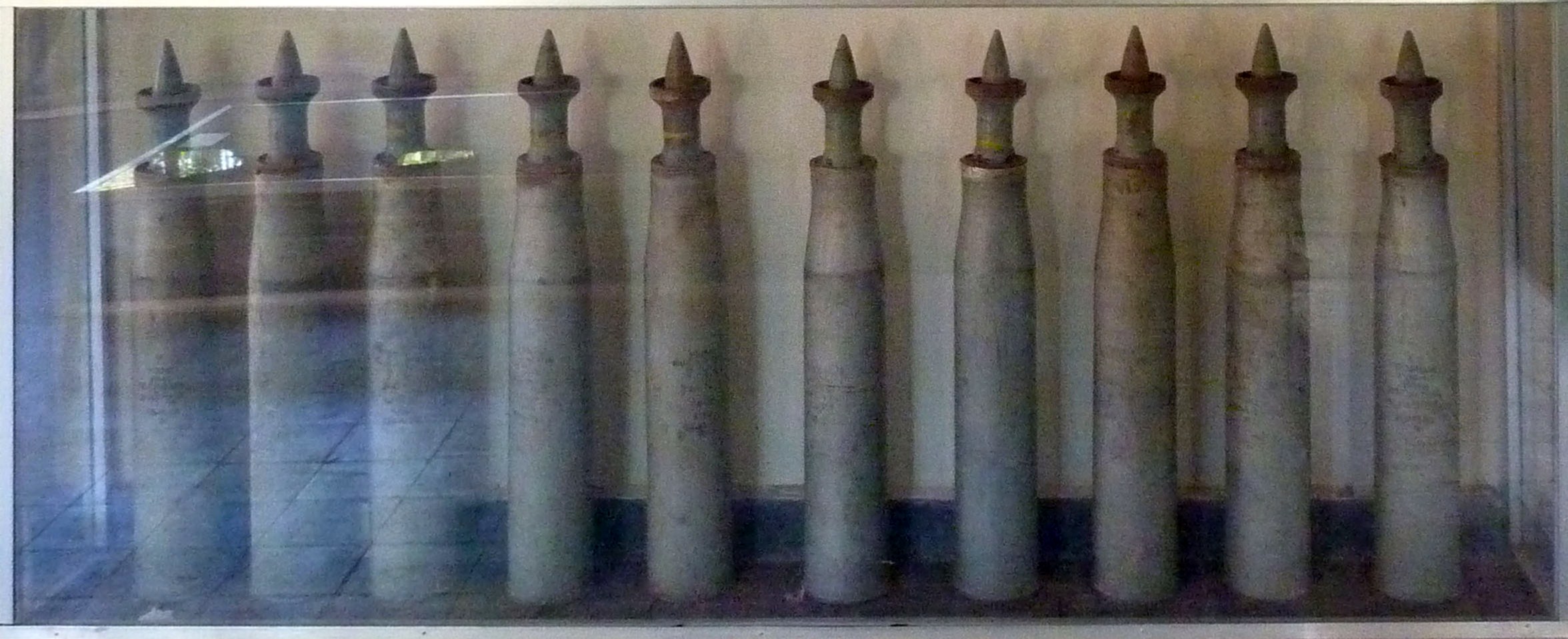This image displays a set of ten large, silvery, metallic objects that resemble bullets, bombs, or some kind of ordinance. They are neatly arranged in a row within a glass case featuring reflective surfaces that slightly obscure the view with glimpses of possible background elements like trees or wooden boards. The objects are all uniform in size and design, each having a tubular base that tapers into a conical top, culminating in a sharp, spiked tip. The back wall of the case is a whitish-brown color, while the bottom shelf is dark brown, contrasting with the silver-toned objects. There is also a noticeable dark blue border at the base of the display. Some of the objects appear to have a rusted or brownish-copper hue around the conical section, possibly indicating either rust or dirt. The glass casing itself is trimmed with silver, adding to the polished appearance of the display.